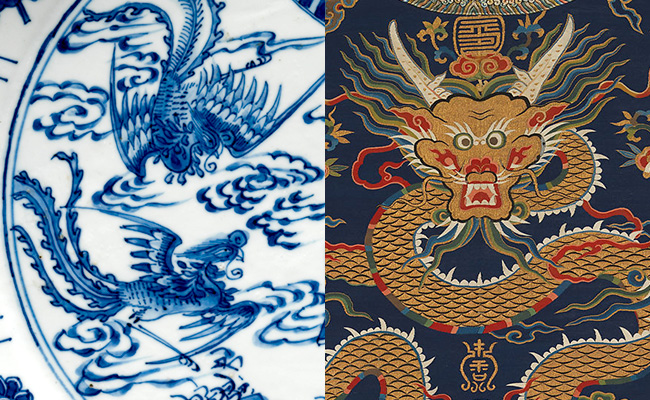The image displays two side-by-side color photographs showcasing intricate Asian artwork. The left photograph features hand-painted blue and white porcelain china adorned with mythical phoenix figures. The phoenixes are depicted with large feathered wings, ribbon-like tail feathers, and intricate swirling patterns surrounding them. The right photograph presents a detailed fabric tapestry with a central golden Chinese dragon. The dragon boasts light-colored horns, blue and green hair or tentacles, and scales that shimmer in gold against a dark blue background. Its snake-like body and caricature-like face with open mouth convey a dynamic energy, further emphasized by the Chinese characters embroidery.